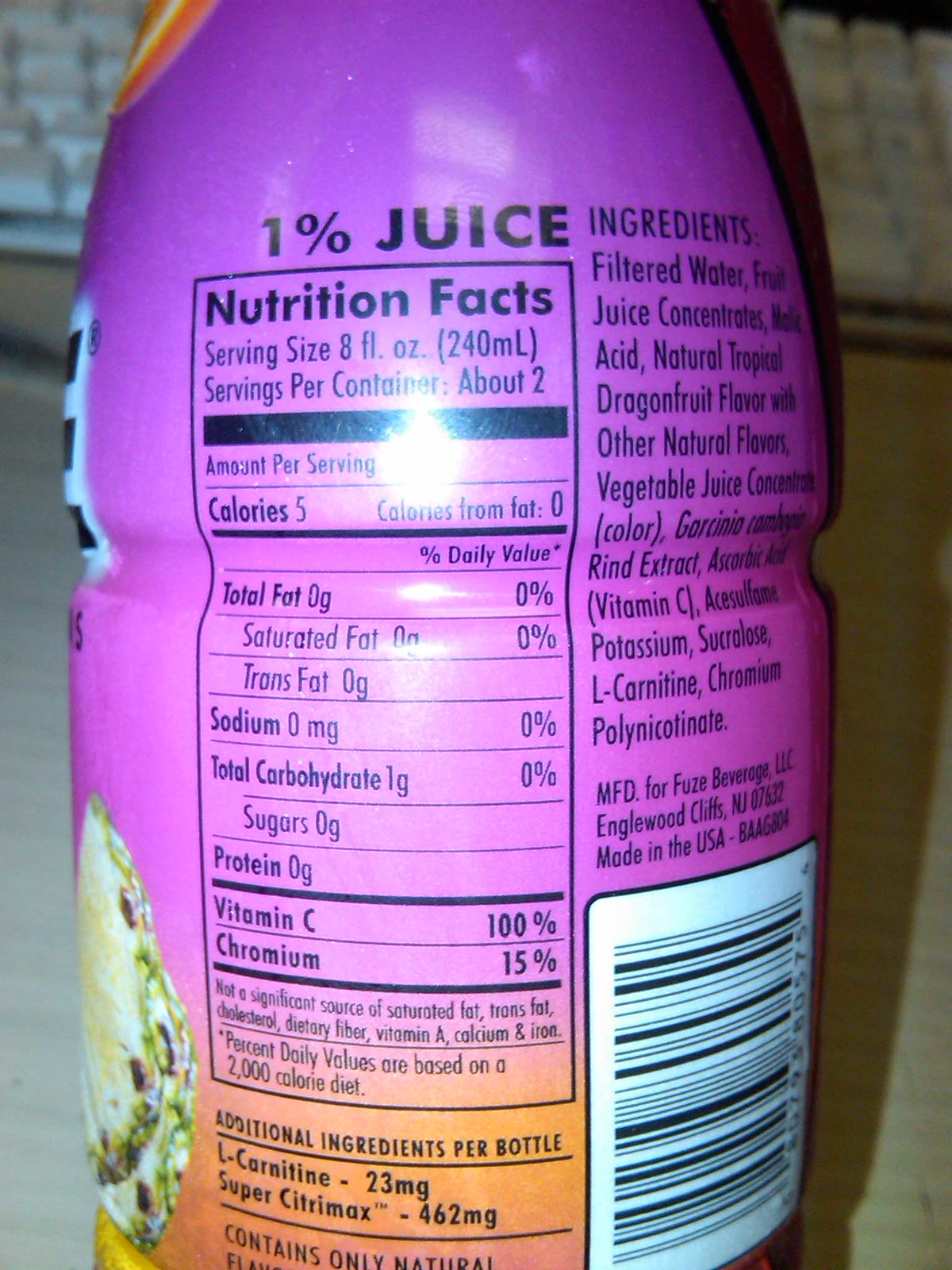Photograph of a vibrant, multi-colored bottle of flavored drink set against a warm, tan background. In the backdrop, a white keyboard can be subtly seen, though the bottle remains the focal point. The bottle features a striking gradient design, transitioning from purple at the top to orange at the bottom. On the left-hand side of the label, there's an image of a pineapple, indicating the flavor. Detailed information is clearly displayed on the label, including ingredients such as 1% juice, filtered water, fruit juice concentrate, malic acid, natural tropical dragon fruit flavor, vegetable juice concentrate, garcinia cambogia rind extract, ascorbic acid, potassium sucrose, l-carnitine, and chromium polynicotinate.

Nutritional facts specify a serving size of 4 ounces, with about 2 servings per bottle, each containing 5 calories and 0 calories from fat. The label indicates 0 grams of total fat, saturated fat, trans fat, and sodium. There is 1 gram of carbohydrates but 0 grams of sugars and proteins. The drink boasts 100% of the daily recommended intake of vitamin C and 15% chromium. A bright light illuminates the bottle, creating a reflection that highlights the nutritional information section.